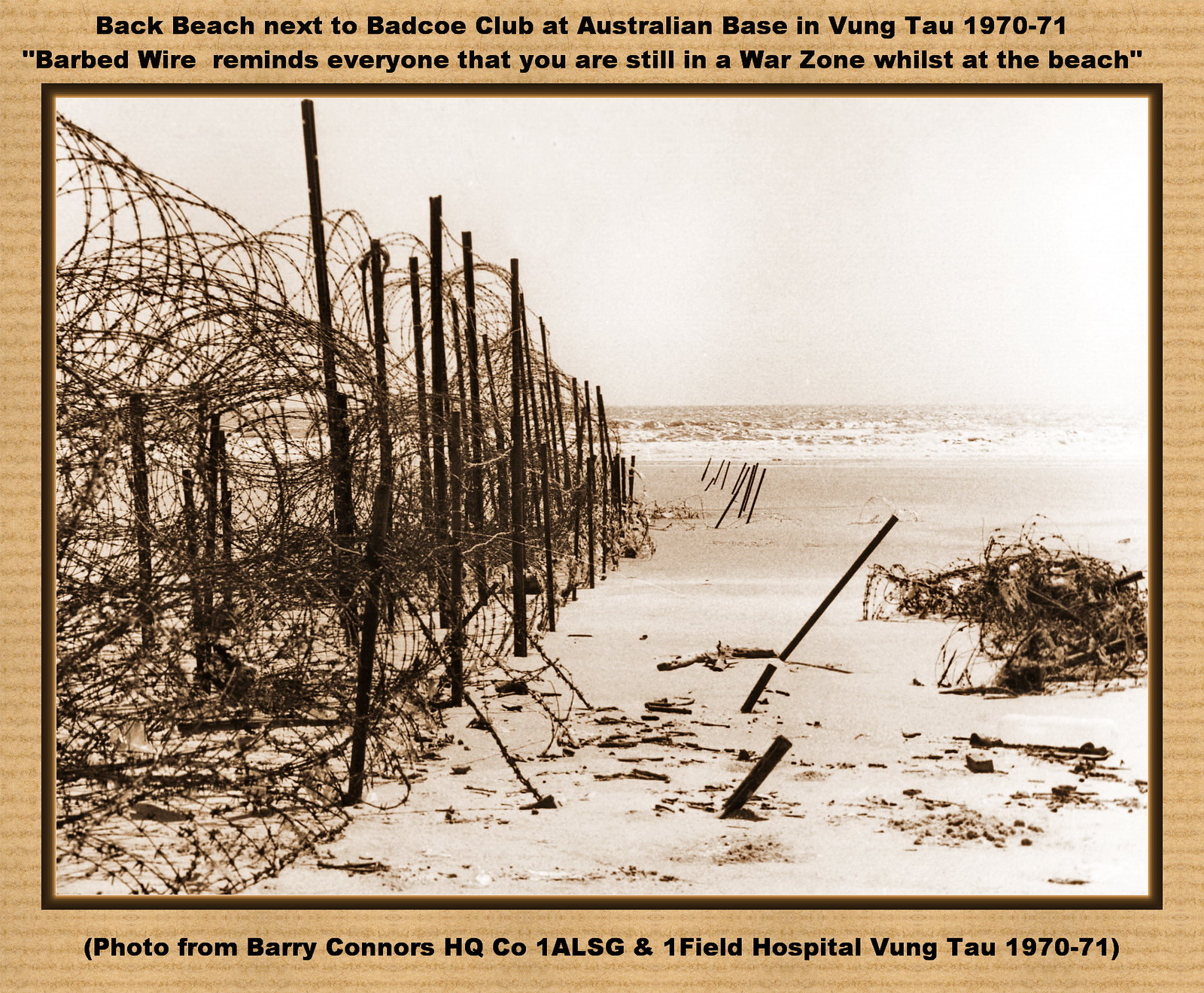This almost sepia-toned photographic image captures a beach scene at an Australian base in Vung Tau during 1970-71. Dominating the foreground is a striking ensemble of rusted stakes and tangled barbed wire, forming a stark barrier along the beach. In the distance, the ocean stretches out under a gray sky, reinforcing the somber mood. Debris is scattered across the sand, adding to the desolate atmosphere. The photograph is set within a dark brown border, adding an additional layer of somberness. Text at the top of the image reads, "Back Beach next to Bad Co. Club at Australian Base in Vung Tau, 1970-71. Barbed wire reminds everyone that you are still in a war zone whilst at the beach." Below the photo, more text reads, "Photo from Barry Connors, HQ Co., 1 ALSG and 1 Field Hospital Vung Tau, 1970-71," crediting the source of this evocative snapshot of life during wartime.